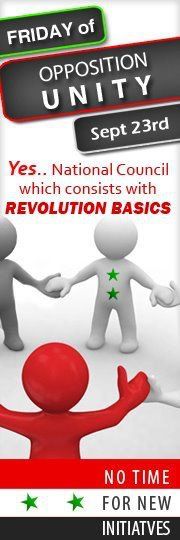The image is a flyer with a white background and several detailed elements. At the top of the flyer, there are three black boxes aligned to the left. The first box, surrounded by a green border, reads "Friday of"; the second box, with a red border, states "Opposition Unity"; and the third box, enclosed by a white border, indicates the date "September 23rd." Below these, in red text, it says, "Yes National Council which consists with Revolution Basics."

The central part of the flyer features three play figures that resemble the Pillsbury Doughboy. They are holding hands, symbolizing unity. The middle figure is white with two green stars across its chest. To the front is a red figure, and another white figure can be seen to its right. At the bottom of the flyer, there is a descending tricolored stripe: red, white, and black, with green stars in the white section. The phrase "No Time for New Initiatives" accompanies this stripe.